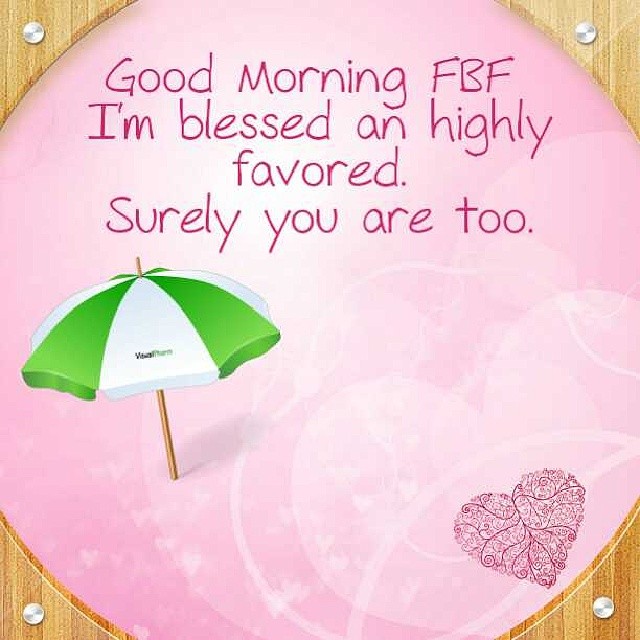This image appears to be a digitally designed graphic, likely intended for social media, featuring a message and illustrations. The focal point is a large, cropped pink circle at the center, decorated with delicate, lacy heart designs, including a dark pink heart with swirling lines resembling leaf veins in the bottom right corner. The text within this circle, written in dark pink, reads: "Good Morning FBF. I'm blessed and highly favored. Surely you are too." To the left of the text, there is a green and white striped beach umbrella with a tan wooden pole. The entire design is set against a background that mimics light pine-colored wood, complete with shiny nails or rivets at each corner, emphasizing the handcrafted, rustic aesthetic of the graphic.